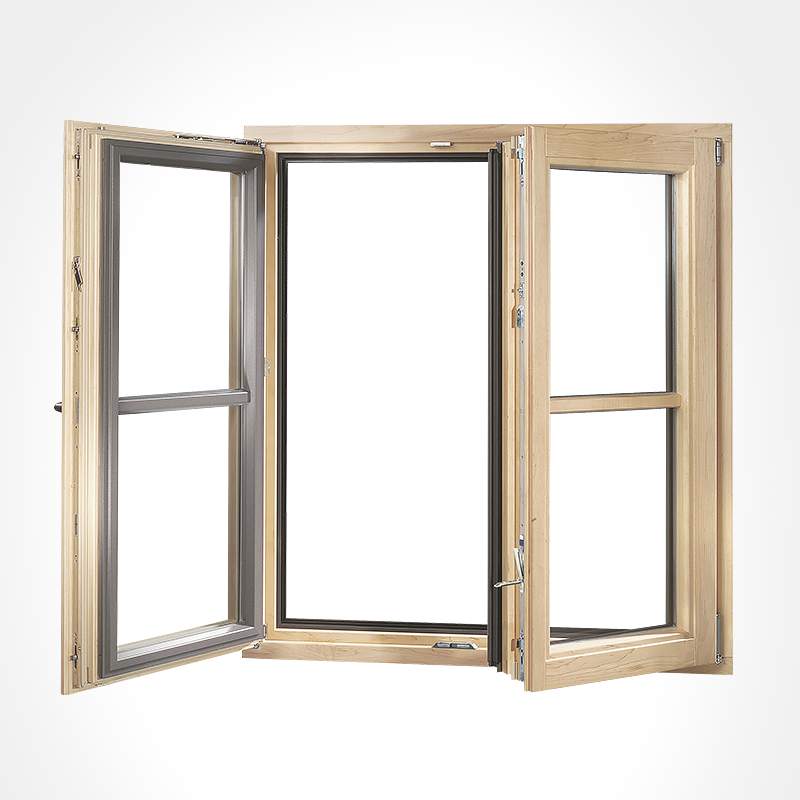This image features a detailed rendering of a wooden-framed window set against a solid white background. The light brown wood frame, which is reminiscent of a shade similar to pine, encloses two main window panels that can both open outward towards the viewer. The window is designed with a central dividing wooden board, allowing each side to hinge and expand independently. The right panel is fully opened, while the left is partially ajar. Both panels are composed of double panes with narrow sections visible and include a line separating each of the two sections. The image showcases silver hinges and a black rubber stopper that help align and seal the windows when closed, preventing air from passing through. This suspended, out-of-context view focuses on the intricate details and mechanisms of the window itself, highlighting its aesthetic and functional design elements.